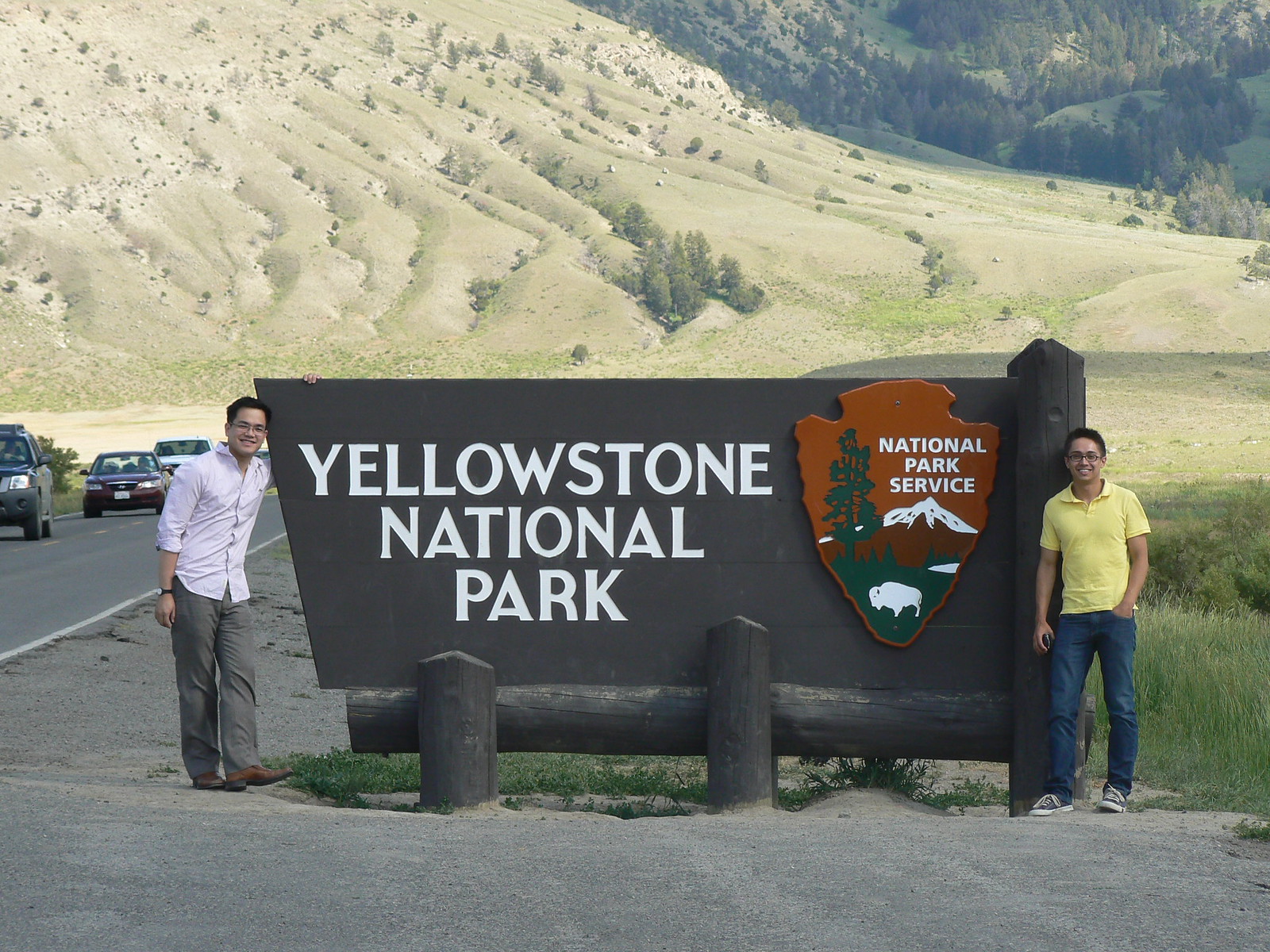In this photograph, two Asian men are standing beside a large wooden sign for Yellowstone National Park. The sign, a massive structure made of dark timber with a nearly gray appearance, features "Yellowstone National Park" in bold white letters. To the right of the text, there is an arrowhead-shaped emblem for the National Park Service, depicting a mountain, a tree, and a buffalo. The two men flank the sign; the man on the left wears black glasses, a white button-down shirt, gray pants, and brown shoes, while the man on the right also sports black glasses, a yellow polo shirt, blue jeans, and black sneakers. Behind them, a scenic backdrop of grassy, tree-dotted mountain ridges unfolds. The scene includes a road along which cars are visible, moving towards the photographer. It’s a striking image capturing both the grandeur of Yellowstone's landscape and a moment of human connection.